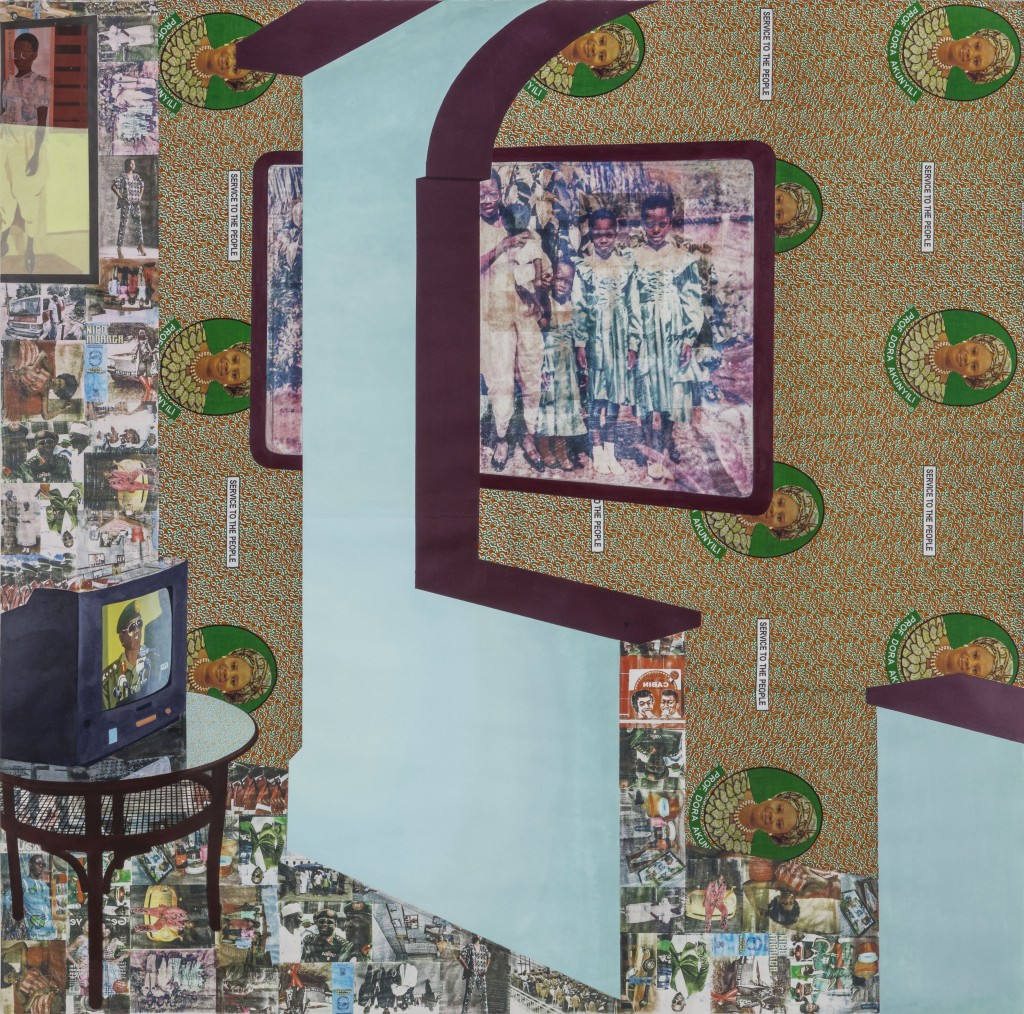This vertical rectangular image titled "Backyard Opera" by Najika Akinya-Crosby features an intricate collage composed of various layered elements, seamlessly blending to create a detailed indoor scene. The dominant background consists of brown wallpaper applied sideways, showcasing vertical oval pictures — one of which prominently features an older African-American woman — interspersed with unreadable text strips. On the right side, a wall segment with an archway stands out, presenting a complex view akin to peering through a window, exhibiting a painting in a purple frame amidst colorful layers of cutouts and figures, predominantly African-American individuals.

Dominating the left-hand side is a small television set situated on a circular glass table supported by brown wooden legs. The surrounding floor and walls are densely covered with various magazine covers and pictures, extending from the left edge downwards. This artwork evokes a mosaic feel through its jumbled yet harmonious incorporation of diverse photographs and cutouts, juxtaposed against a vivid tapestry of backgrounds, making this scene come to life with intricate details and cultural depth.